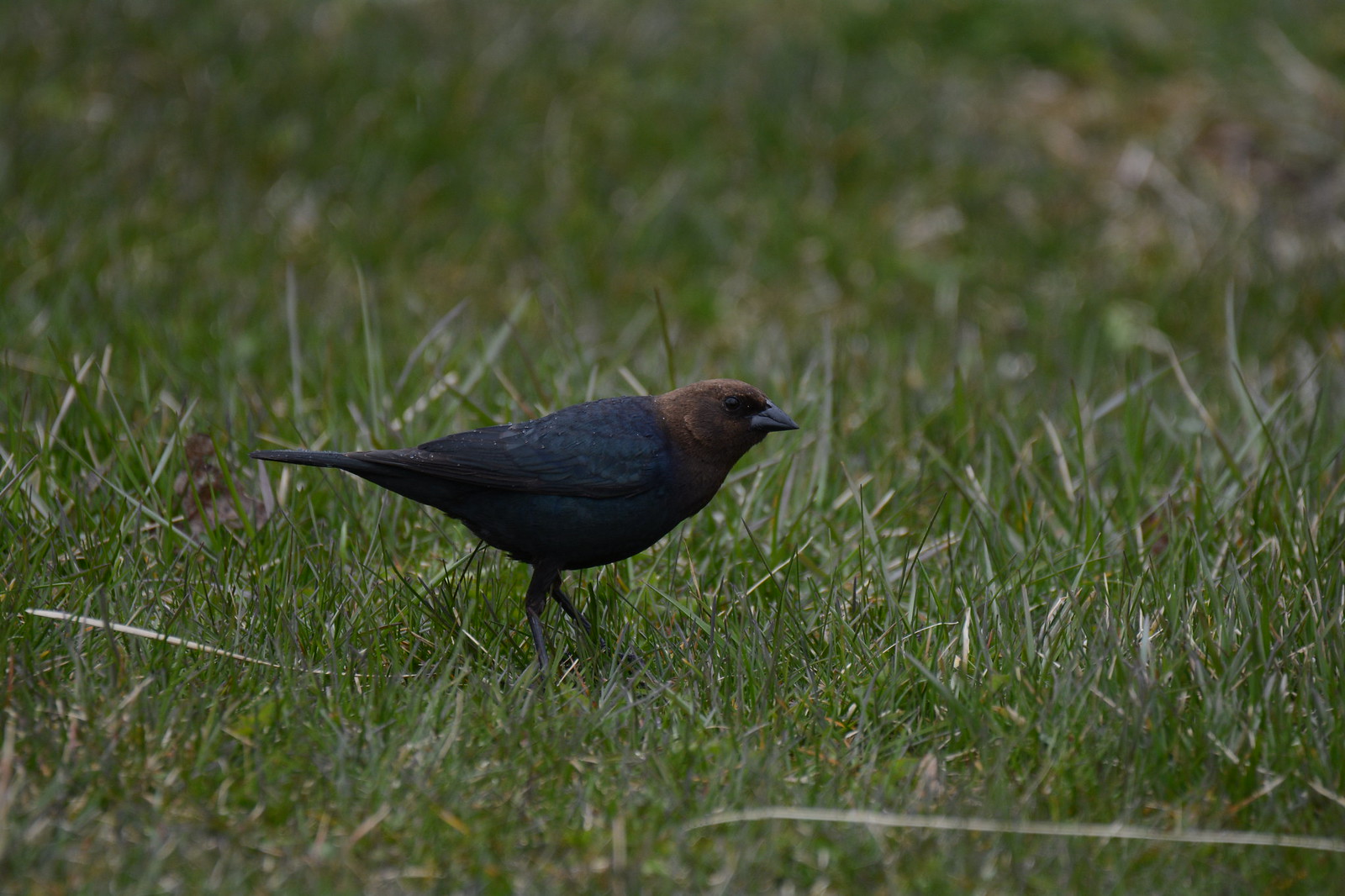A striking close-up image captures a black bird walking through a patch of thick, wild grass. The bird’s body is predominantly black with a shimmering iridescent blue on its wings and upper body. Its head is a dark brown, complemented by a short, dark beak. Only parts of its black legs are visible as its feet are obscured by the dense grass. One leg slightly leads the other as it strides from left to right. The bird’s tail features a mix of green and dark blue feathers. Its eyes are a glossy black.

The grass surrounding the bird is mostly vibrant green, interspersed with a few yellow and white blades, hinting at a whimsical, untamed nature of the field. The background is beautifully blurred, keeping the bird as the central focus of the image. In the bottom right corner, a long yellow blade of grass stretches from the right edge to the center of the image, laying flat on the ground. Near the bird, a dark brown leaf lies nestled in the greenery, adding to the rustic feel of the scene.